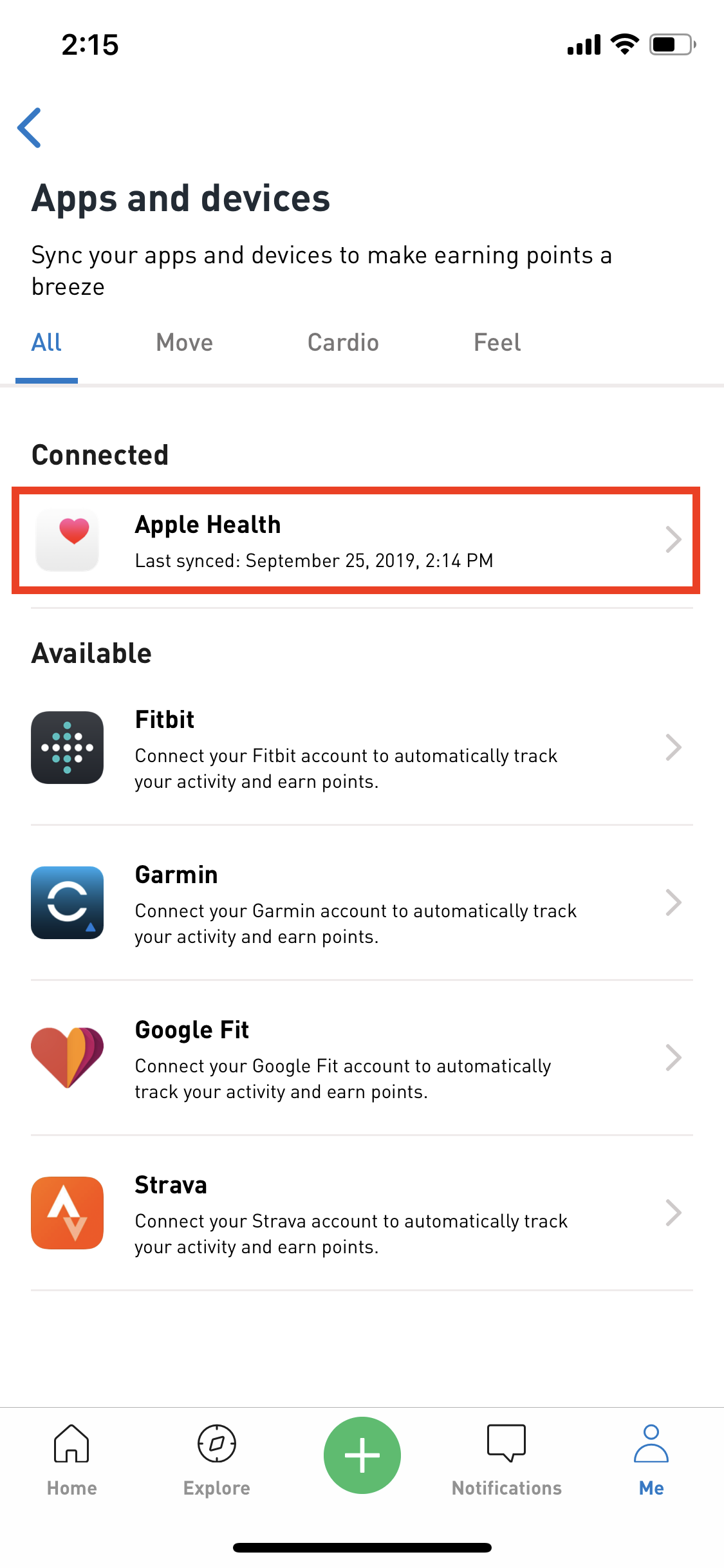The screenshot displays a mobile app interface at 2:15 PM. At the top, the header reads "Apps and Devices" in bold black text. Below, a prompt encourages users to "Sync your apps and devices to make earning points a breeze." The user has selected the "All" tab, which is underlined in blue, alongside options for "Move," "Cardio," and "Feel."

Under the header "Connected," the first connected app is Apple Health, marked with a heart icon to the left. It shows the last sync time as September 25th, 2019 at 2:14 PM, with an arrow icon to the right for more information. The selection is highlighted with a red border, indicating it is actively being viewed or managed.

Other available options include Fitbit, Garmin, Google Fit, and Strava. Each option comes with a brief description: for Fitbit, “Connect your Fitbit account to automatically track your activity and earn points,” similarly echoed for Garmin and Google Fit. Fitbit features a small icon illustrating the brand.

At the bottom of the screen, a navigation bar contains icons labeled Home, Explore, a Plus button, Notifications, and Me, with the "Me" section currently selected, highlighted in blue. The entire interface is designed to facilitate effortless syncing of fitness and health tracking apps, promoting a seamless experience in monitoring and earning points for physical activities.